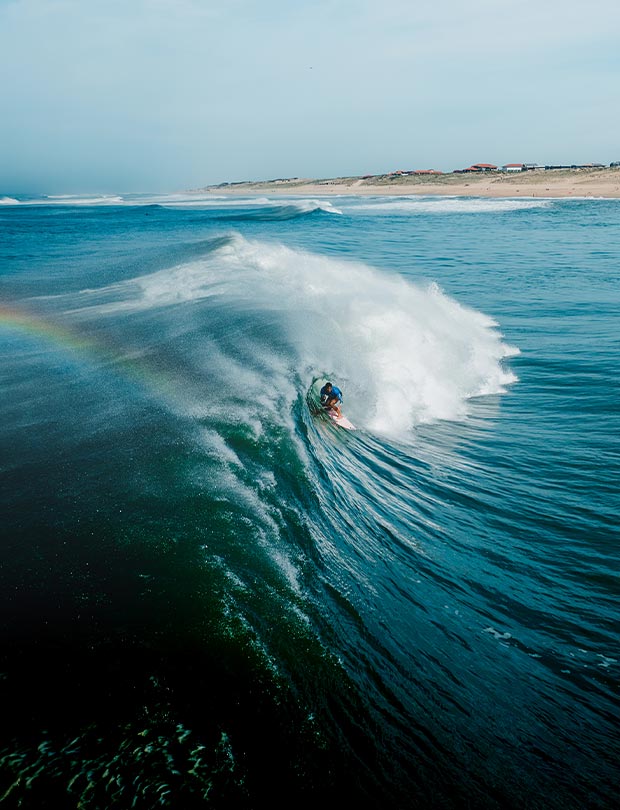This captivating image showcases a surfer expertly catching a large wave in the ocean. The surfer, dressed in a blue and black wetsuit, is crouched down on a pink surfboard as the wave crests with white foamy tops. On the left-hand side, a vibrant rainbow arcs gracefully, adding a burst of color to the scene. The water beneath is a deep bluish-teal, and in the lower left-hand corner, a school of fish is visible at the base of the wave. The backdrop reveals a beach with some red-roofed buildings, set against a cloudy, greyish-blue sky that hints at impending rain, contributing to the vintage feel of the photograph. The sun is obscured by clouds, casting a soft, diffused light over the entire scene.